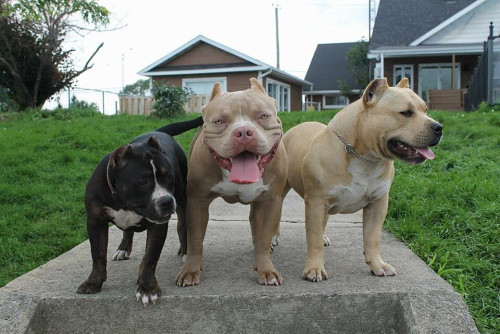This color photograph, captured in landscape orientation, vividly features three bulldogs situated at the top of a set of concrete steps in what appears to be a backyard. The central figure, a tan and white bulldog, stands prominently with its mouth open, displaying the characteristic pant of its breed, and gazes directly at the viewer with an almost daring expression. To its left, a smaller black and white pup with a white muzzle, chest, and paw looks slightly to its right, aligning its view with its companions. On the right side of the image, another light brown, or tan, bulldog with rounded ears and a white chest, glances off to its left. Behind the trio, an unkept lawn of green grass stretches towards two well-maintained houses visible in the background, which appear painted and in good condition. The photograph, captured under a gray sky, bathes the scene in soft light, contributing to the comfortable demeanor of the dogs, despite the overcast weather. The rich details and photorealistic style offer a candid and engaging glimpse into a moment in the lives of these young canine guardians.